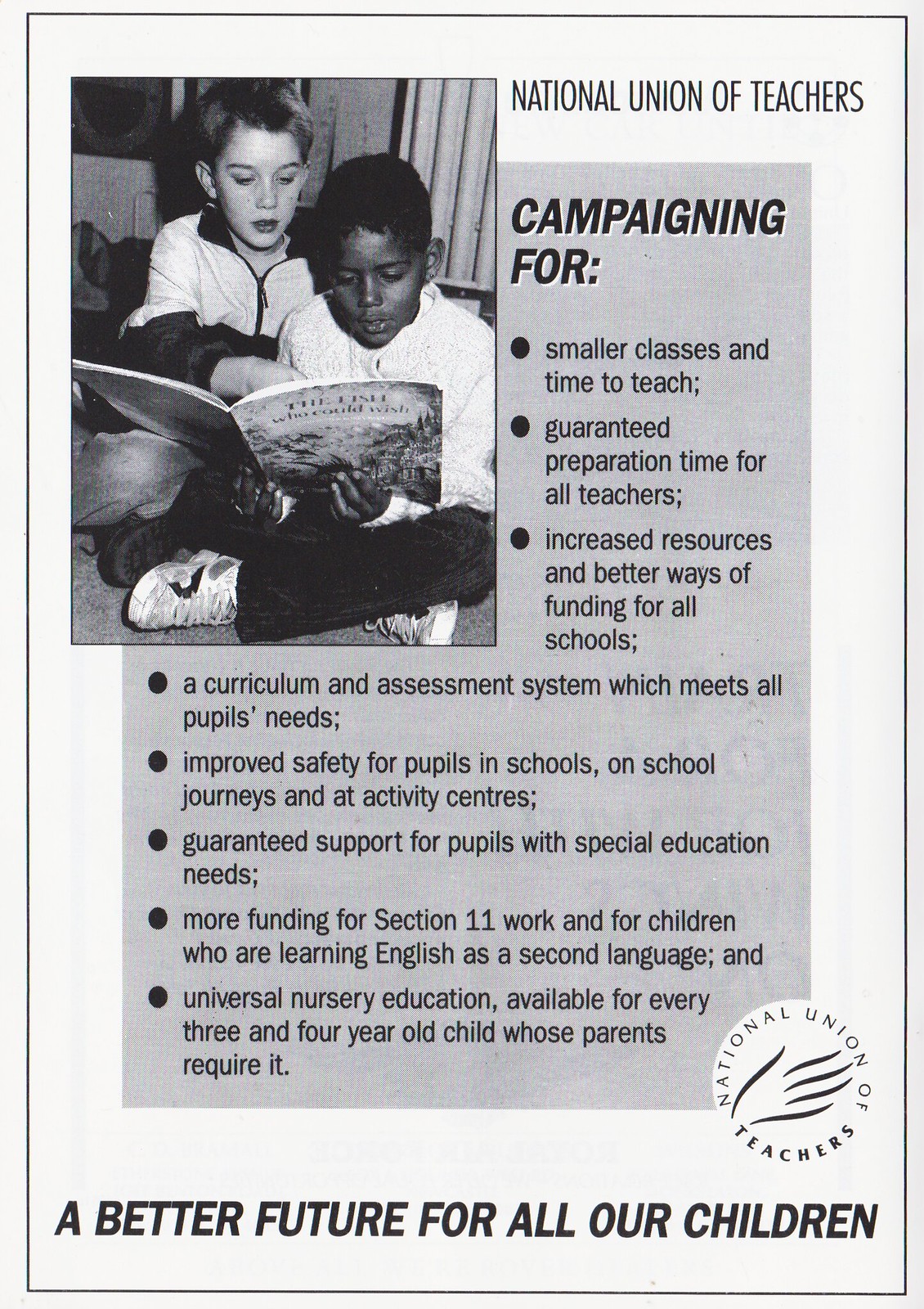The poster from the National Union of Teachers, set against a very light blue background, features a photograph in the top left quarter of two young boys sitting cross-legged and engrossed in a children's book. The African-American boy, approximately eight years old, is holding the book and wearing a white shirt with dark pants and white shoes featuring black details. Beside him, a Caucasian boy, of similar age, is sitting just behind to the left, looking down and pointing at the book. He is dressed in a white zip-up sweater with black accents.

Adjacent to the photograph, the text "NATIONAL UNION OF TEACHERS" is prominently displayed in black uppercase letters. Below this title, set within a gray rectangular section with a thin white frame, the poster lists various campaign points in black uppercase letters under the heading "CAMPAIGNING FOR." The bullet points include:

- Smaller classes and time to teach
- Guaranteed preparation time for all teachers
- Increased resources and better funding for all schools
- A curriculum and assessment system which meets all pupils' needs
- Improved safety for pupils in schools, on school journeys, and at activity centers
- Guaranteed support for pupils with special educational needs
- More funding for section 11 work and for children learning English as a second language
- Universal nursery education available for every child aged three and four whose parents require it

A neatly organized, horizontally aligned series of black oval bullets delineates these points. At the bottom of the poster, within a white oval featuring a simple line drawing of a hand, the text "NATIONAL UNION OF TEACHERS" is repeated, with "A BETTER FUTURE FOR ALL OUR CHILDREN" inscribed in large black uppercase letters across the bottom. This detailed and organized design, reminiscent of the 1960s, emphasizes the call for educational reforms aimed at creating a better future for all children.